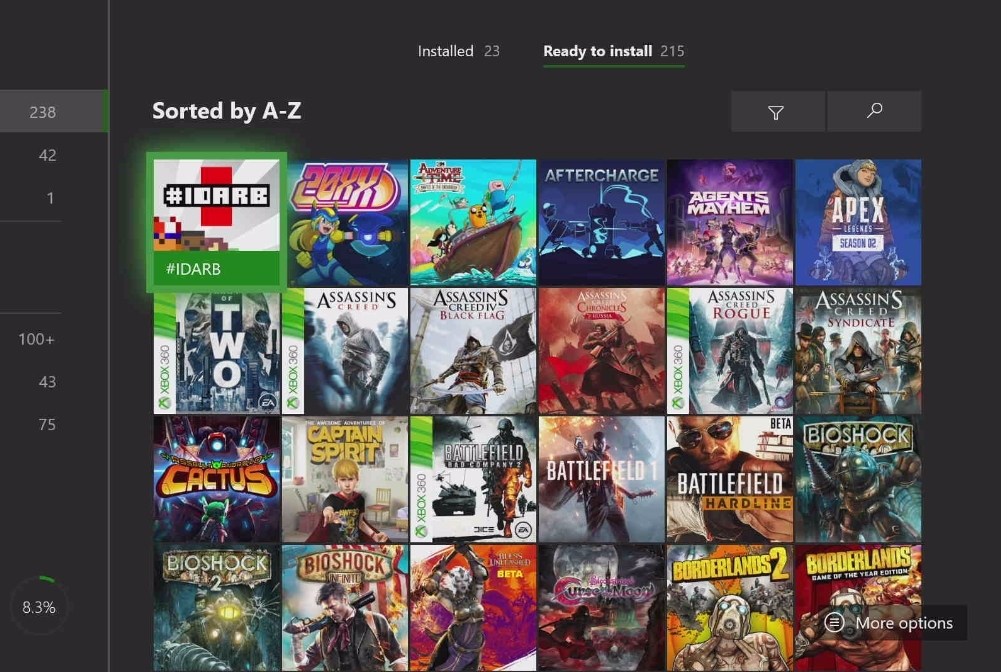The image is a detailed screenshot of a gaming console interface, specifically displaying an Xbox 360 library. At the very top, in white text, it states "Installed 23, Ready to Install 215," with "Ready to Install 215" underlined in green, indicating the current selection. 

To the left side of the screen, there are vertically aligned numbers: 238, 42, and 1, with 238 in a light gray bar, a gap, then "100+," 43, and 75. 

The main section in the middle features a dark gray background populated with game titles, organized alphabetically from A to Z. The games are displayed in large rectangular blocks. 

The first row reads: IDARB (highlighted with a green border that slightly obscures the game underneath), 20XX, Adventure Time, Aftercharge, Agents of Mayhem, and Apex Legends Season 2.

The second row continues with: an obscured title, Assassin's Creed, Assassin's Creed IV Black Flag, Assassin's Creed Chronicles: Russia, Assassin's Creed Rogue, and Assassin's Creed Syndicate.

The third row includes: an obscured title (partially covered by the game "Cactus"), The Awesome Adventures of Captain Spirit, Battlefield: Bad Company 2, Battlefield 1, Battlefield Hardline, and BioShock.

The fourth row lists: BioShock 2, BioShock Infinite, a title possibly reading “Bless Unlimited Beta”, Cursed Mood, Borderlands 2, and Borderlands: Game of the Year Edition.

Towards the bottom right of the screen, there is a rectangular button labeled "More Options," accompanied by a circle featuring three horizontal white lines.

This image captures the expansive gaming library available on this particular Xbox 360 console.